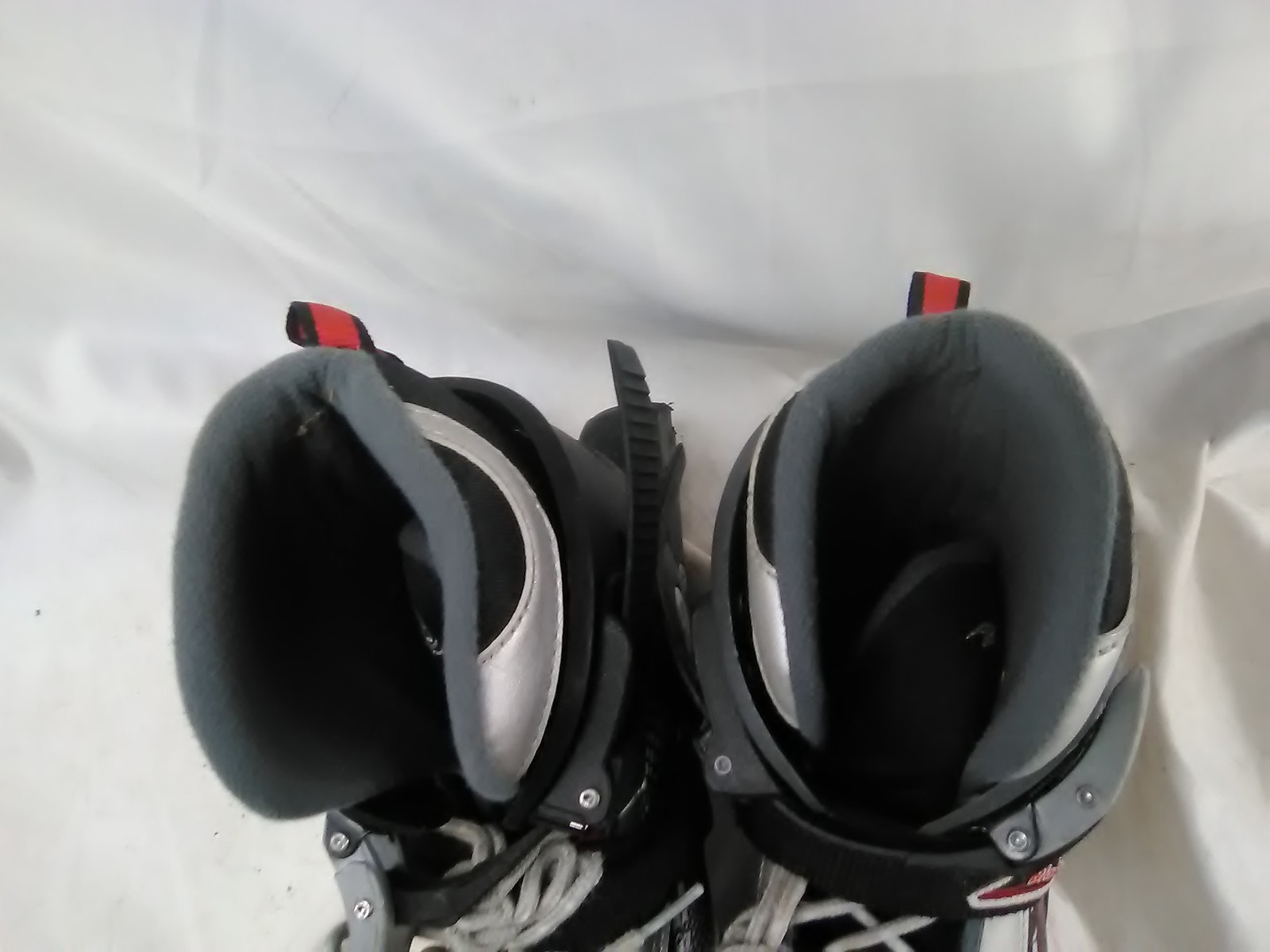This is a color photograph capturing a close-up, top-down view of a pair of roller skates set against a smooth, greyish-white cloth background. Each skate features a roundish, breathable black fabric exterior with white stitched accents, including white laces and a distinctive white stripe. The interior of the skates, where you would insert your feet, is a gray material. On the back of each skate, there is a small, red and black-edged ribbon. The left skate's bindings are open, while the right skate's bindings are locked closed. The skates, positioned side by side, occupy about three-quarters of the image's width, and the cloth beneath them appears creased, particularly under the right skate. Enhanced lighting toward the lower right-hand corner of the frame highlights the intricate textures and details of both the skates and the fabric.